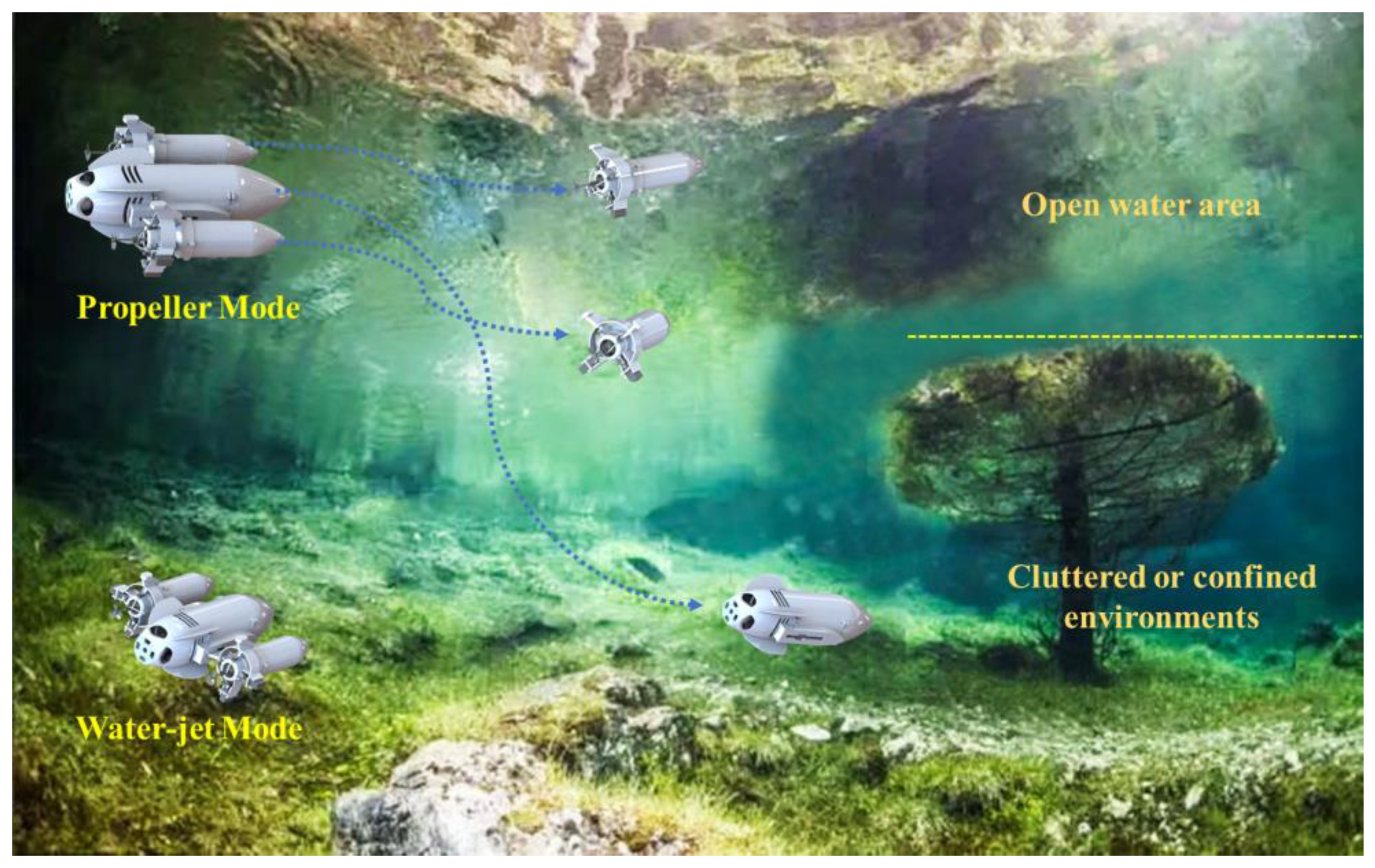An underwater rendering showcases a proposed undersea unmanned exploration vehicle in both propeller and water jet modes. The vehicle, positioned on the left-hand side of the image, consists of a central pointed cylinder flanked by two smaller autonomous sub-vehicles. The image illustrates these sub-vehicles being launched from the main craft, with dotted lines depicting their separation paths. In the background, an underwater cave environment is visible, characterized by an algae- or seaweed-covered floor and what appears to be a tree. The area is divided into an "open water area" at the top right, illuminated by light from an opening above, and a "cluttered or confined environment" around the tree. The central cylinder is shown exploring the cluttered area while the sub-vehicles head toward the open water region. Text annotations in yellow highlight the different modes and environments within this aqua-hued scene.